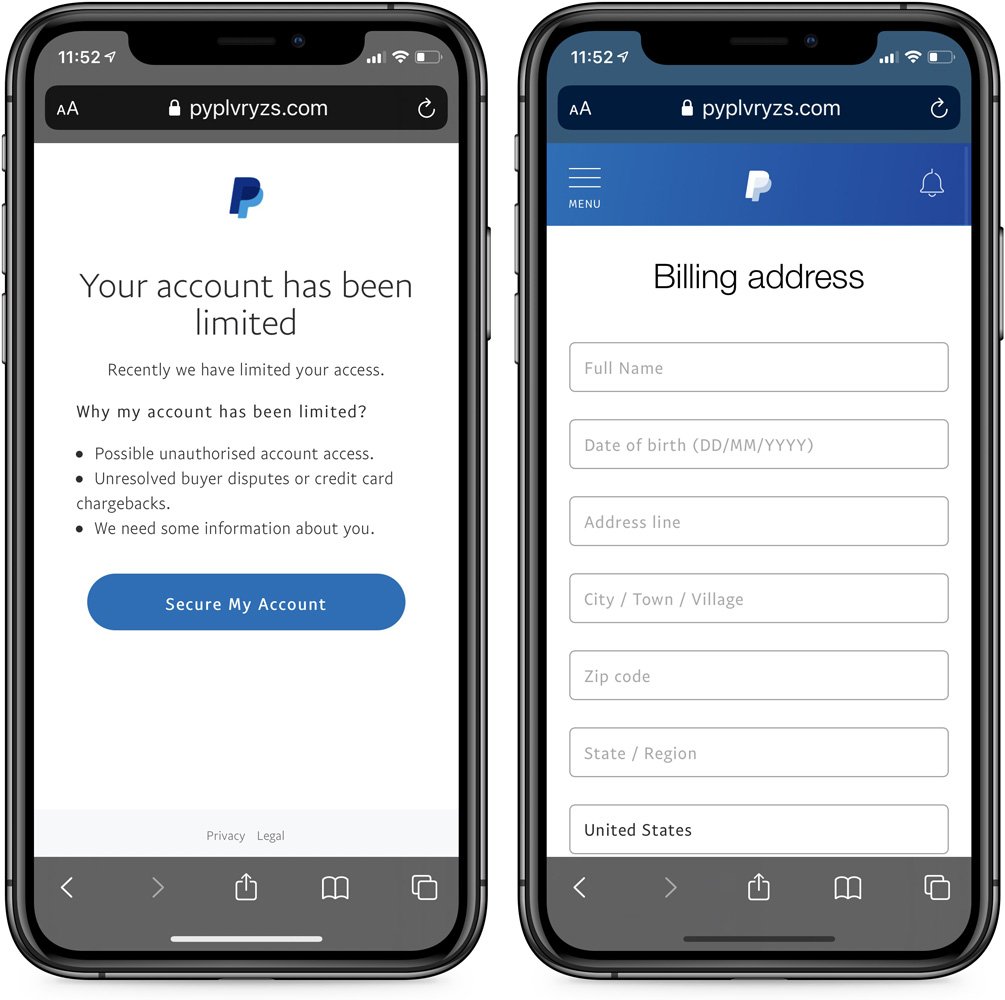This is a detailed description of two screenshots displayed side-by-side on cell phones. The first screenshot shows a PayPal account alert stating "Your account has been limited". The user is informed that their access has been restricted and is provided with a large blue button to "Secure Your Account". This screen lists the reasons for the account limitation and the steps needed to resolve it. 

The second screenshot, displayed on the second cell phone, shows another PayPal page requesting the user's billing address information. There are multiple input fields outlined with thin gray lines and pre-filled with light gray placeholder text. The fields ask for details in the following order: "Full Name", "Date of Birth" (with a specified format), "Address Line", "City, Town, or Village", "Zip Code", "State or Region", and finally, "United States", which is already filled in and displayed in black font.

These screens are presumably being referenced on a third device not shown in this image.